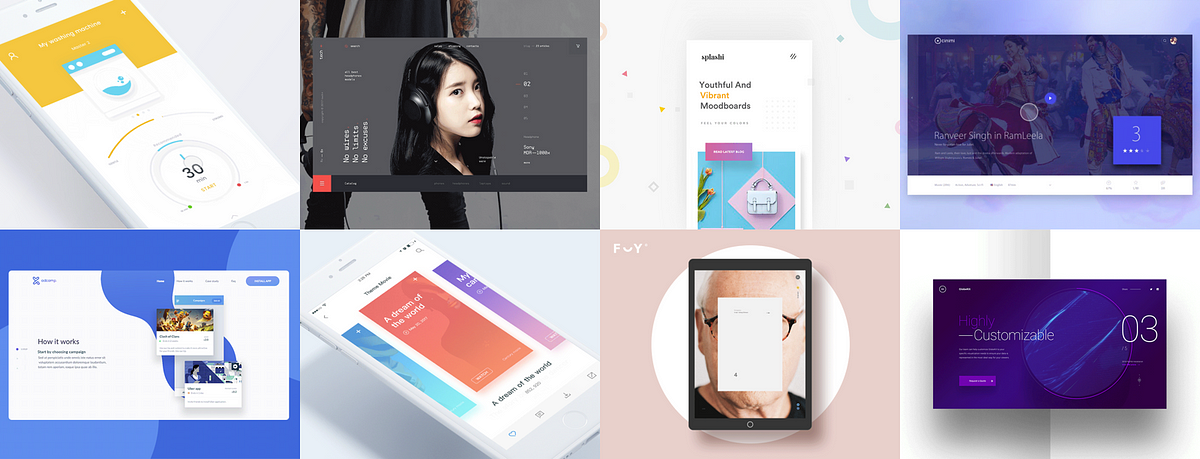This composite image showcases a mix of various pictures and graphics, possibly sourced from multiple devices or a website. The first section depicts a potential iPhone displaying the number 30 within a circle, suggestive of a measurement app. Overlaid on this is a computer-generated icon resembling a washing machine.

Adjacent to this, on the right, there's a portrait of an Asian woman with long black hair and headphones. She stands to her left while subtly peeking to her right, set against a gray backdrop.

Further to the right is an image bearing the word "useful," accompanied by what appears to be a phone icon and a purse graphic. This is followed by a predominantly blue-toned picture, featuring faded sports figures and text, with the number three prominently displayed within a blue box.

Below this, a segment titled "how it works" is positioned on the left, next to an image of a phone. Beside this phone, there's another tablet-like device, likely a non-iPad, displaying a bald individual with their face partially obscured by another image.

On the right side of this composite, an additional image contains the phrase "customizable three."